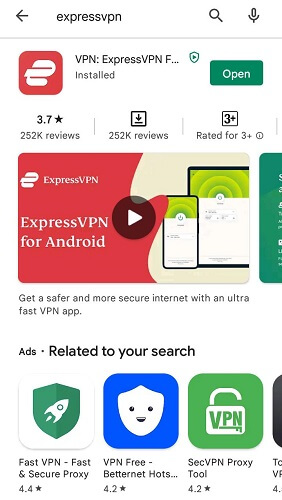The image is a detailed screenshot displaying an application listing on a white background. In the top left corner, there's a left-pointing arrow next to the text "ExpressVPN." Beside it, there's an icon of a magnifying glass and a microphone.

Beneath these icons, a prominent red box with the ExpressVPN logo, characterized by three horizontal white lines, catches the eye. The text next to the logo reads, "VPN, ExpressVPN installed." A green rectangle below this text states, "Open," indicating the app is installed and ready to launch. Below the green rectangle, there is a rating of "3.7 stars" based on "252k reviews," and the app is rated for users aged "3+."

Further down, a video with a play icon in the center displays, captioned "ExpressVPN for Android." The video showcases both a phone and a tablet, presumably displaying ExpressVPN's home page. Under this visual, a descriptive sentence promises, "Get a safer and more secure internet with an ultra fast VPN app."

Finally, at the bottom in bold black letters, it says "Ads related to your search." Below this, there are three icons with an ad for a different app labeled "Fast VPN, fast and secure proxy," which boasts a rating of "4.4 stars."